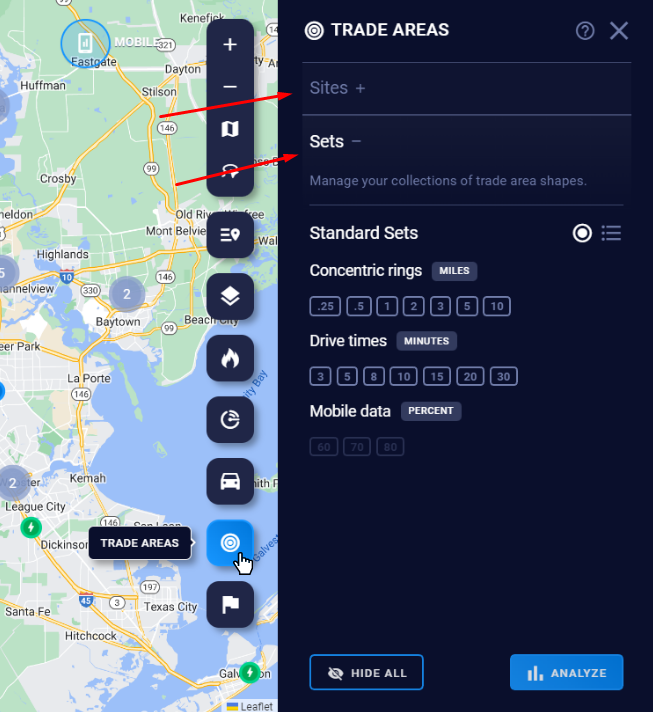A detailed caption for the image described could be:

---

A detailed map interface displaying various tools and options. On the left, the main map features highways and marked locations. On the right, an array of icons allows for map interaction, including zoom buttons (+ and -), an information icon, a flame icon, a circular icon, a car icon presumably indicating drive times, and a flag icon. The highlighted icon with a hand/pointer is labeled "Trade Areas". To the right of "Trade Areas", a section with a red arrow labeled "Sites +" is positioned at the top, and below it another red arrow points to "Sets", stating "Manage your collection of trade and area shapes." Below that, a "Set Standards" section details options like concentric rings for distances ranging from 0.25 to 10 miles, drive time in minutes, and mobile data. At the interface's bottom, options to "Hide All" or "Analyze" are available, hinting that the tool is designed to assist salespeople or professionals in analyzing geographic data and trade areas.